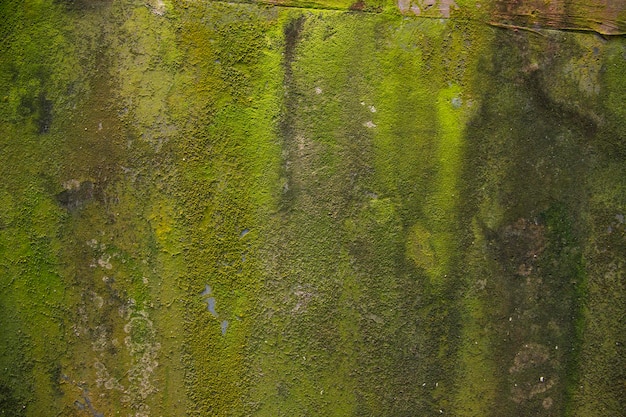This image portrays a highly textured, abstract scene dominated by varying shades of green, suggesting a natural or possibly artistic representation. The surface features a range of green hues, from neon to dark, intertwined with black slashes and brown coloring, primarily on the right side. White speckles sporadically dot the image, resembling either chipped paint or reflections of light on a mossy or muddy surface. The upper portion of the image reveals a crack, with a wood-like texture seen above it, enhancing the organic feel. From an aerial perspective, this could be interpreted as a marshy land covered in dense, low grass or moss, with small pockets of water interspersed throughout. The straight lines of green running down contribute to the overall structured, yet abstract, presentation of the landscape.